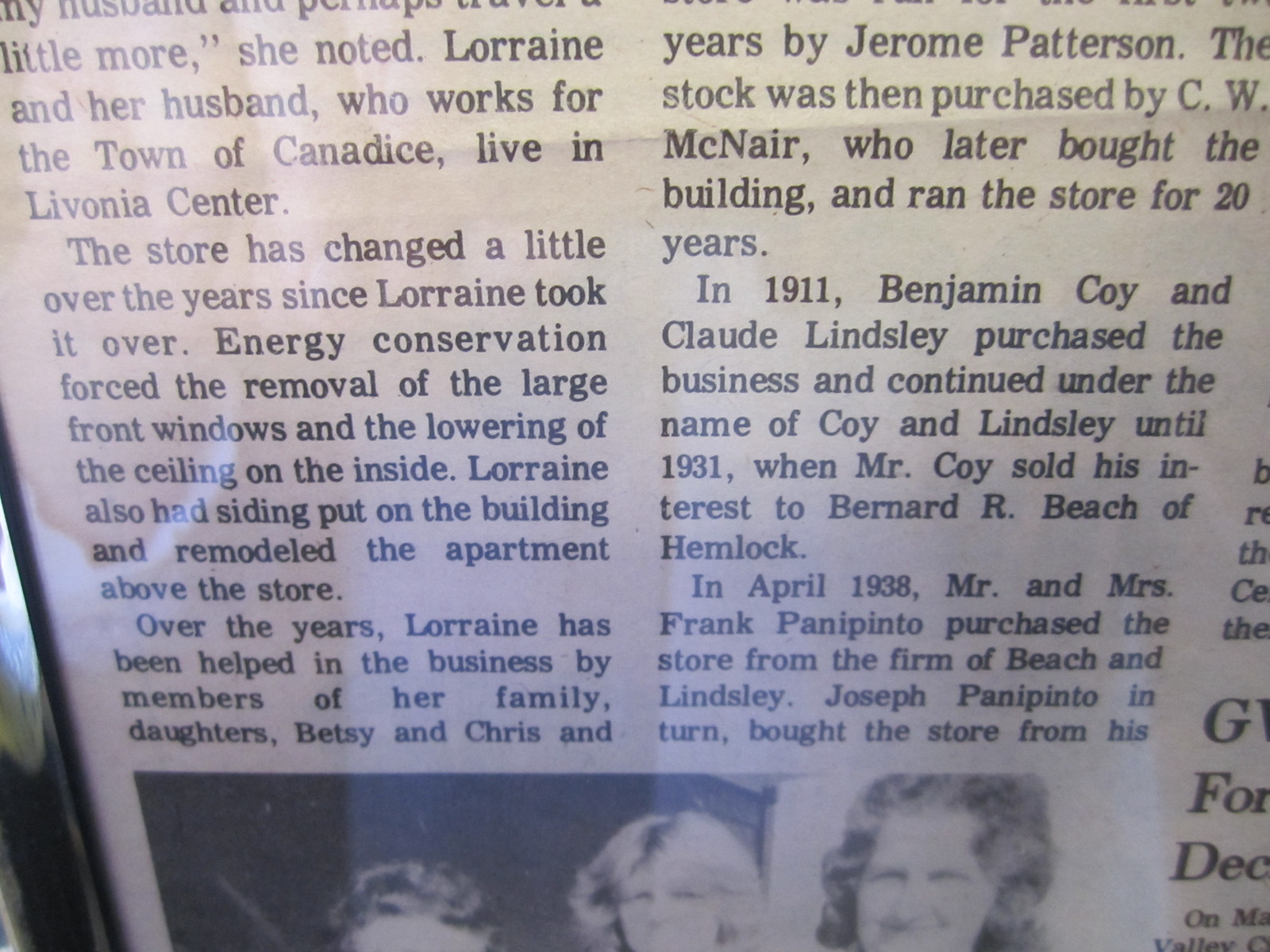The image captures a close-up photograph of a framed newspaper clipping, which is enclosed behind glass, evidenced by a subtle reflection on the surface. The visible portion of the article spans two main columns of text, with only a small part of a third column. Featured at the bottom of the clipping is a black-and-white photograph of three women, possibly Lorraine and members of her family, reflecting the article’s subject matter. 

The partial text that can be read details a story about Lorraine and her family, who run a longstanding store in Livonia Center. The text begins with, "Little more," she noted, "Lorraine and her husband, who works for the town of Canadas, live in Livonia Center. The store has changed a little over the years since Lorraine took it over. Energy conservation forced the removal of the large front windows and the lowering of the ceiling on the inside. Lorraine also had siding put on the building and remodeled the apartment above the store. Over the years, Lorraine has been helped in the business by members of her family, daughters Betsy and Chris."

The narrative continues with historical context about past ownerships, mentioning several individuals including Jerome Patterson, C.W. McNair, Benjamin Coy, Claude Linsley, Bernard R. Beach, and the Ponipinto family, who have been associated with the store from its inception up until various transfers of ownership. The article gives a glimpse into the evolution of the store and its community relevance over the years.